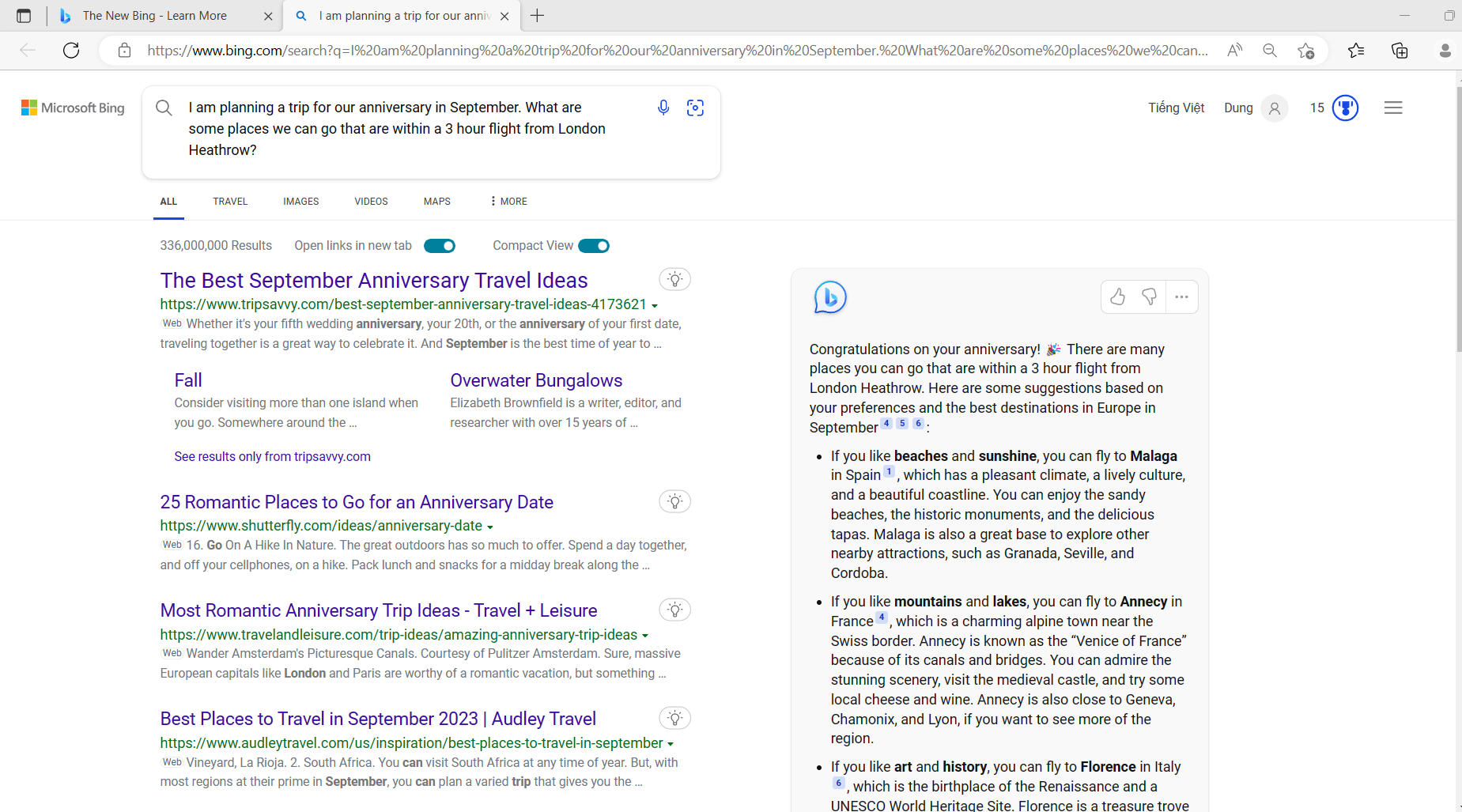A screenshot of Microsoft Bing's interface is displayed. The top section features a dark gray border. In the left corner, there is a thickly outlined black square, slightly thicker at the top. Next to it, the blue Microsoft icon is visible, followed by the text in black that reads "the new Bing, learn more". Adjacent to this text, a blue search icon displays the phrase "I'm planning a trip for A-N-N" which appears to be cut off. 

Directly below this, there's a search bar containing "bing.com," followed by an extended series of numbers. In the left section of this area, a small square is comprised of mini-squares in red (top left), green (top right), yellow (bottom right), and blue (bottom left). To its right, the text reads "Microsoft Bing".

Beneath, a light rectangular box with a search icon on the left highlights a query: "I am planning a trip for anniversary in September. What are next on some places we can go within the three hour flight from London? Heathrow?" Following this, there are six clickable tags.

Displayed search results appear in purple titles, each accompanied by green links directly below. Two lines of detailed black text provide additional information beneath each title. 

On the right side, a light blue pop-up tab is visible. The top left of the tab features a circle with a Bing icon, underlined by a paragraph. Additionally, three dots aligned vertically, each indicates a paragraph with approximately six lines of text.